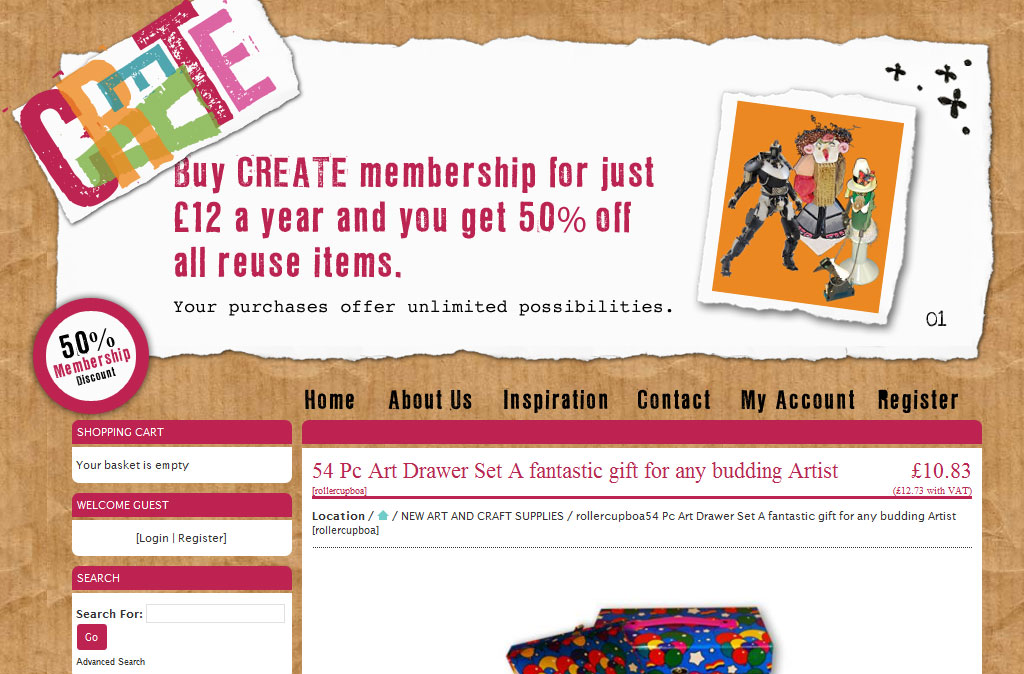The image features a brown background. At its center, there's a tilted square containing the letters C-R-E-A-T-E, arranged haphazardly: the green 'A' lies on its side and the blue 'E' is inverted on top of it. To the left, dark pink text reads, "Buy CREATE membership for just $12 a year and you'll get 50% off all reused items. Your purchase offers unlimited possibilities." 

To the right of this text, a small orange square showcases different characters including a robot and a character with brown hair and a red mouth. Below this, a white text inside a pink circle announces "50% membership." Further below, a pink shopping cart icon is labeled with "Welcome guests" and "Search."

To the far right, category options in black text include: Home, About Us, Inspiration, Contact, My Account, and Register. Beneath a long pink line, a highlighted product is a 54-piece art drawer set priced at $10.83, described as "a fantastic gift for any budding artist." Adjacent is a multicolored bag with a pink handle.